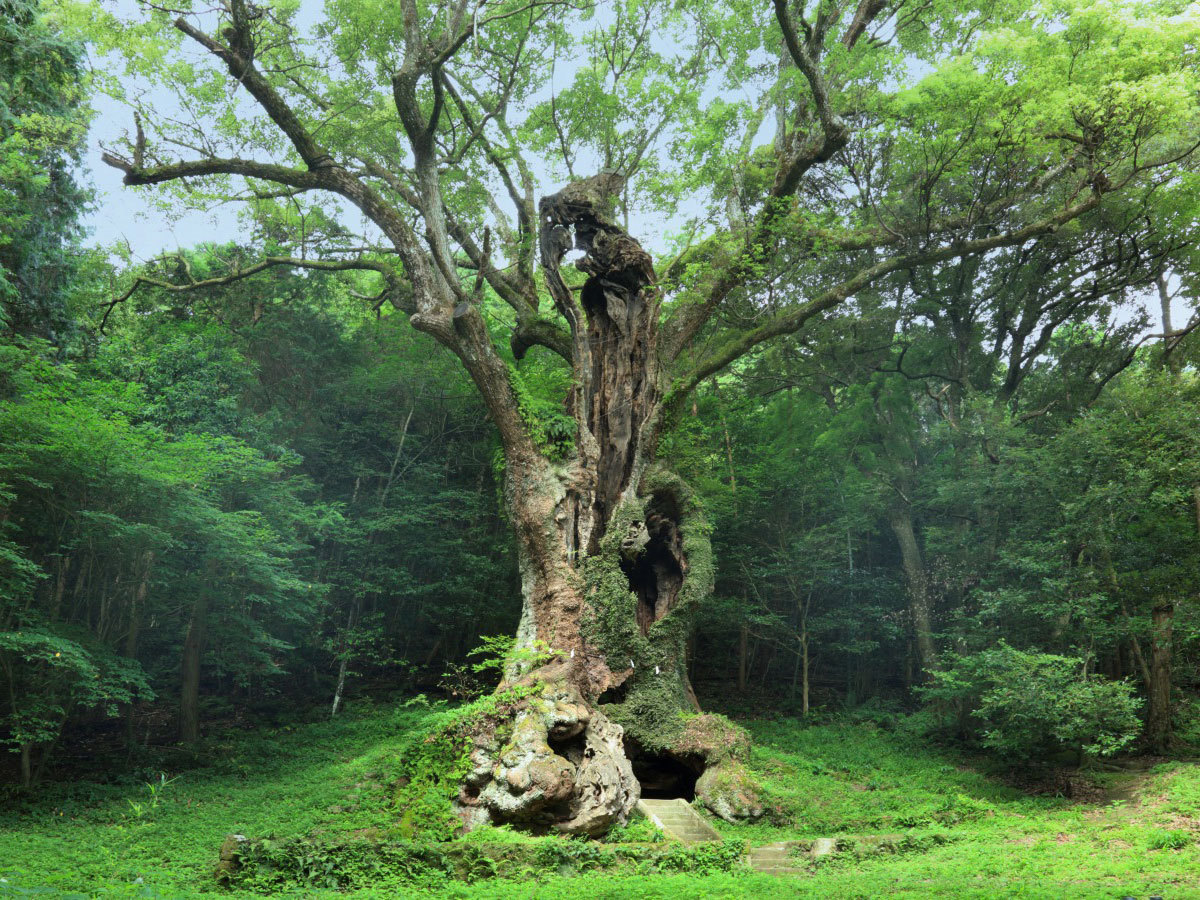In the midst of a dense, seemingly untouched forest, a massive tree commands the scene, its enormous trunk dwarfing the surrounding foliage. The sky above is a mix of blue and scattered clouds, indicating a clear daytime. Nearby trees have leaves ranging from light to dark green hues, contributing to the forest's rich tapestry. The ground is covered in a lush carpet of green grass, but it's the imposing tree that draws the eye. Its sprawling branches extend far and wide, creating an impression of grandeur and dominance. This tree's expansive reach and thick, rugged branches suggest that it has claimed its territory, allowing no other trees to encroach upon its space.